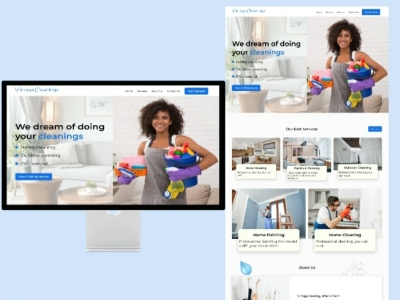This image, sourced from a website, features a predominantly blue background. On the left side of the image, there is a black-bordered rectangle with small, blurry text at the top, which is illegible. Below the text, a photograph of a woman holding cleaning supplies is displayed. Adjacent to this image, the text reads, "We are doing your cleaning," followed by some additional information.
 
Mirroring this section on the right side of the page, there is an identical advertisement, showcasing the same woman with cleaning supplies. The accompanying text reads, "We dream of doing your cleaning." 

Below these advertisements, there are two rows of pictures. The first row consists of two images: one depicting a house and the other, presumably of a garage. The second row contains three images. The first image shows the interior of a house with someone cleaning the walls. The final image on the right captures a person wearing a white shirt and orange gloves, seemingly working on a white cabinet, although their specific task is unclear.